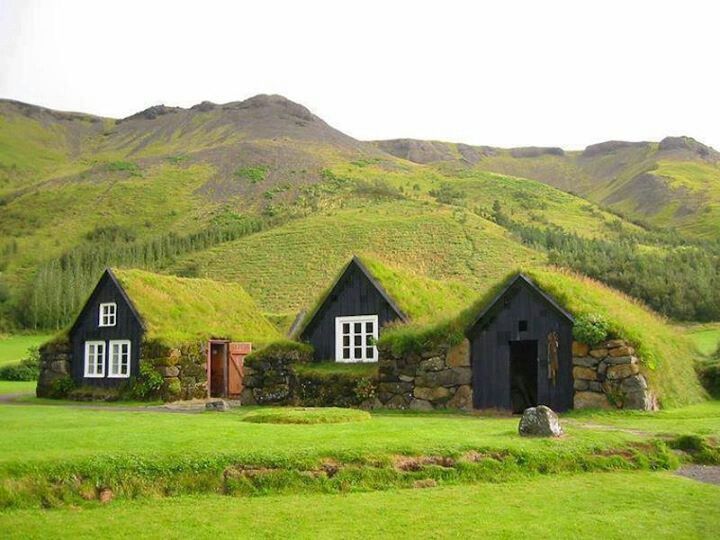The color photograph presents a lush, green hillside adorned with a verdant lawn in the foreground and a white sky overhead. At the foot of the hill, three quaint buildings rest, each displaying a harmonious blend of natural and man-made elements. The structures are intricately crafted with dark, charcoal-colored or black wood, stone walls, and bright white-trimmed windows, contributing to their rustic charm.

The leftmost building features an open wooden door and three distinct white-framed windows—one small at the top and two larger ones below—surrounded by rugged stone and moss-covered walls. The roof, like the hillside, is carpeted with grass, seamlessly blending into the surrounding greenery.

Positioned in the middle, the second building has a simpler design with a single large double window. It shares the same black wood and stone construction, with its roof similarly swathed in lush grass. A grassy ledge in front of this building acts as a natural continuation of the hillside.

The rightmost structure appears to be a shed or barn, distinguished by a small open cutout window above a doorway adorned with what looks like hanging animal skin. This building also features a grassy roof and stone sides. In front of it, a large boulder adds to the rustic landscape.

All three structures nestle snugly against the hill, with green moss and grass embracing their roofs and walls, creating a picturesque, unified scene of nature and architecture. The backdrop showcases green, mossy hills leading up to dark gray mountains, enhancing the idyllic and serene atmosphere.